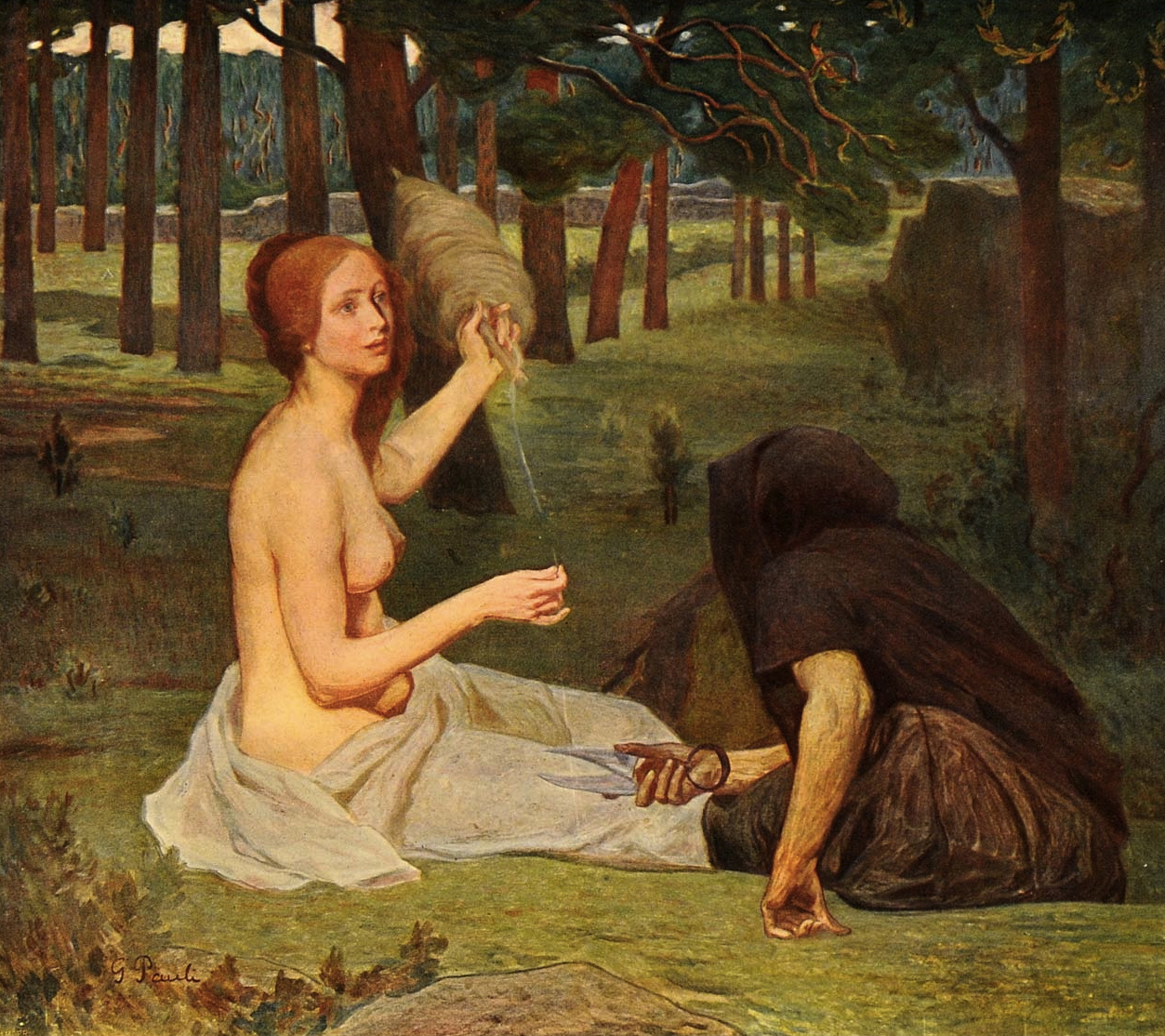This image depicts a detailed, vibrant painting signed with the artist's name "G. Pauli" in cursive at the bottom left. The scene is set in a lush, green forest clearing, capturing a serene yet tense moment. In the foreground, two figures are seated on the grass. The woman on the left is partially nude, draped only in a white sheet around her waist. Her long red hair cascades to her left, with most of it pulled back into a bun. She has a somewhat worried expression, gazing slightly upwards while holding a large spool of yarn on a stick in her left hand, and grasping the end of the thread in her right hand. Across from her sits a dark, enigmatic figure clad in a brown cloak, their hood pulled over their head. This figure, sitting slightly hunched, holds a pair of shears in one hand. The background reveals a picturesque landscape: a field stretches into the distance, bordered by a dense array of trees and rock formations. The contrast between the vibrant greenery and the earth-toned rock formations adds depth to the composition, enhancing the overall tranquil yet mysterious atmosphere of the painting.